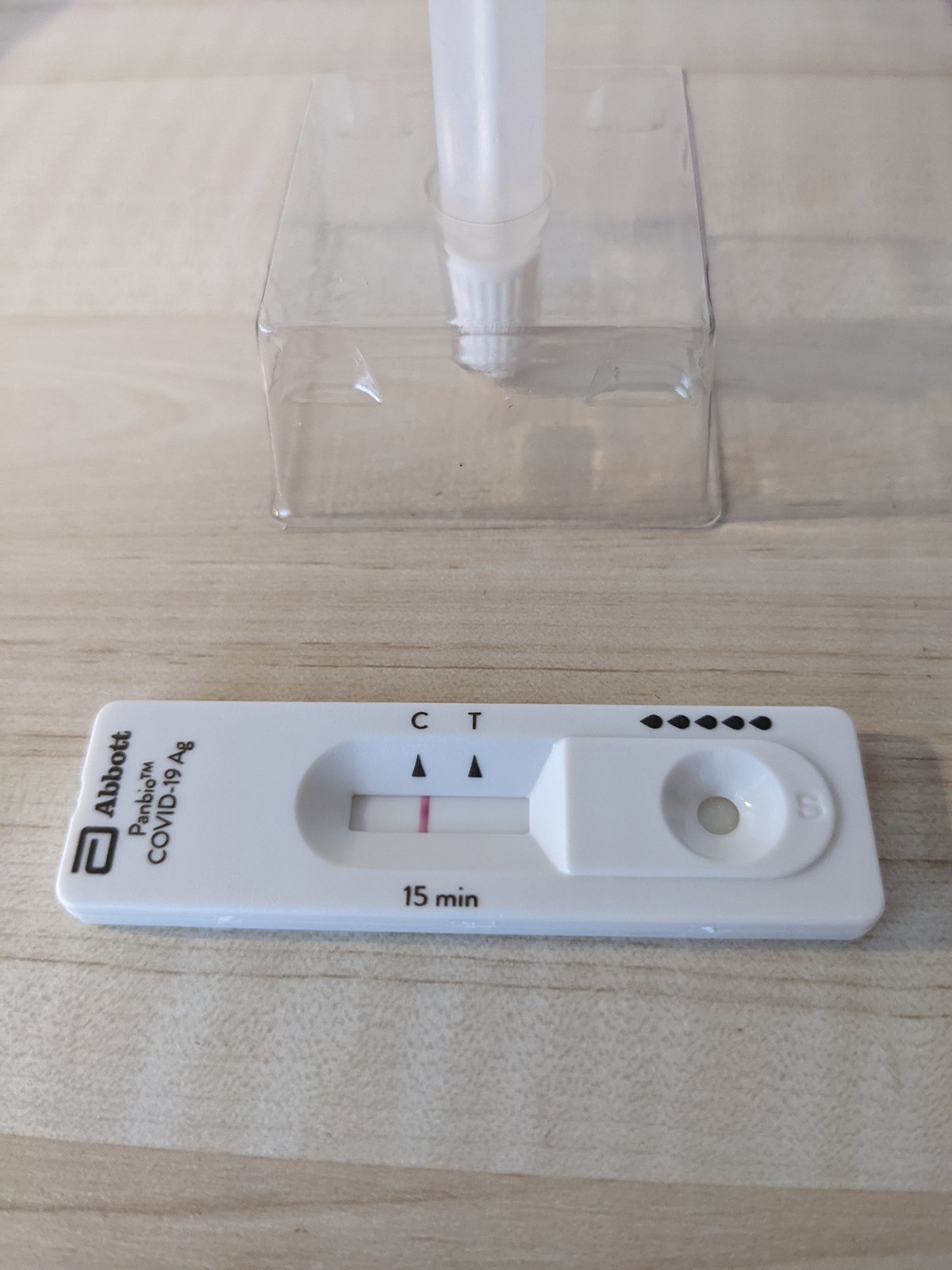On a table with a very light blonde wood stain, the grain clearly visible and accented by whitish stripes, two items are prominently displayed. The first item is a small, rectangular, white plastic COVID-19 test. At the top of the test, "Abbott" is printed in black, followed underneath by "PanBioTM" and then "COVID-19 AG." Along the bottom side of the test, "15 minutes, 15 MIN" is inscribed. A test strip in the middle features a pink line that aligns with the letter "C," which is marked with an arrow beneath it, while the letter "T" also has an arrow pointing to it. At the opposite end of the black print, there is a small round indentation that appears to provide a view of the internal test strip.

A few inches away from the COVID-19 test sits a rectangular glass beaker. Inside the beaker is a small white plastic tube with a white plastic cap. The test and the tube together suggest a thorough and precise setup for administering a COVID-19 test kit.